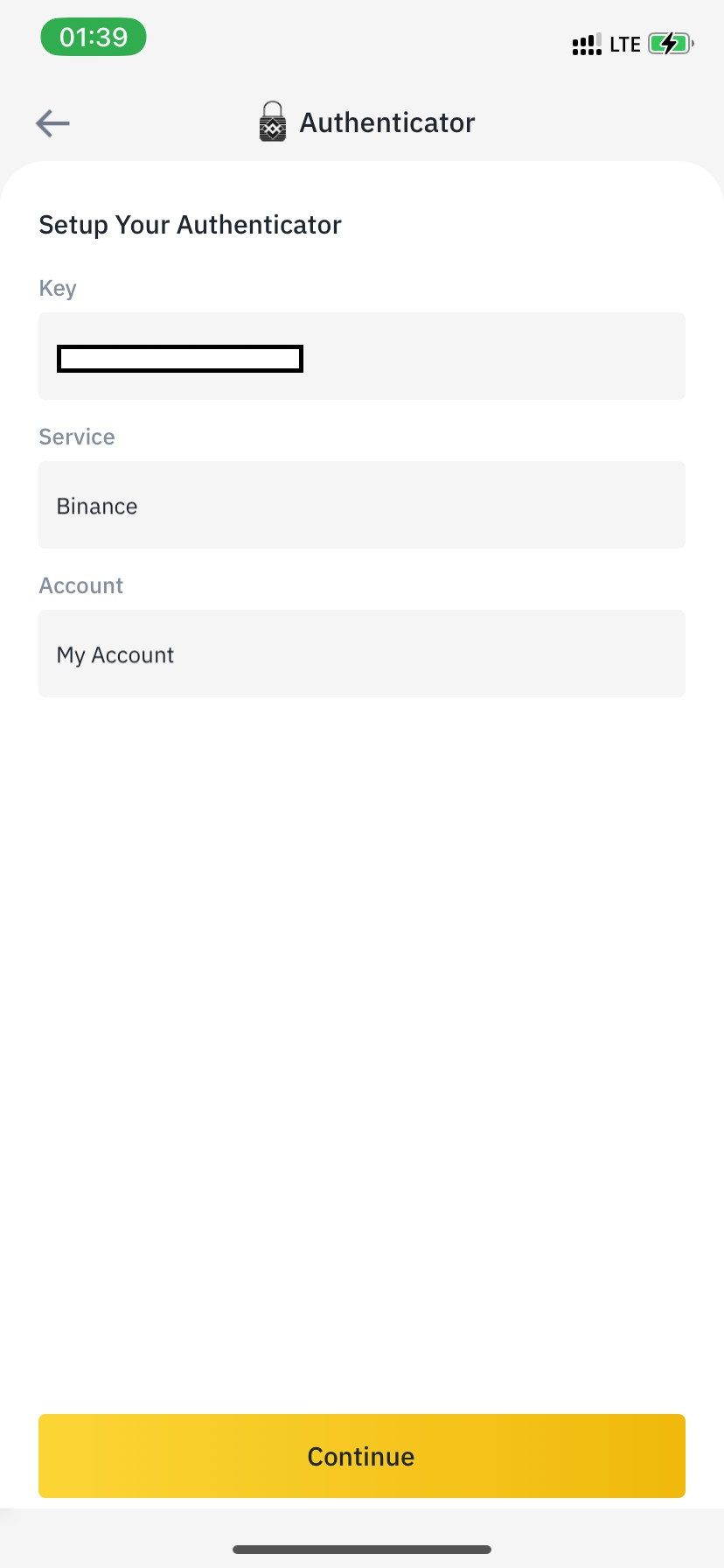The image is a vertically oriented rectangular screenshot of a smartphone display. At the top of the image, there is a gray status bar. On the left side of this bar, within a green oblong shape, the current time "1:39" is displayed in white text. On the right side of the status bar, there are indicators for signal strength (showing LTE connectivity) and a fully charged battery that is currently charging.

Below the status bar, still within the gray area, the word "Authenticator" appears in black text. Accompanying the text, to its left, is a small lock icon and to its right is a left-facing arrow.

The main body of the image falls under a section titled "Set up your authenticator." This section is divided into alternating white and gray areas. It features three main fields: 

1. **Service:** Under this label, the word "Binance" is clearly visible.
2. **Account:** This field displays the text "my account."
3. **Key:** This field is empty but has a black outlined box indicating where the key should be entered.

At the very bottom of the image, an orange button labeled "Continue" is prominently displayed. A gray border, which includes a thin black line, runs along the bottom edge of the image.